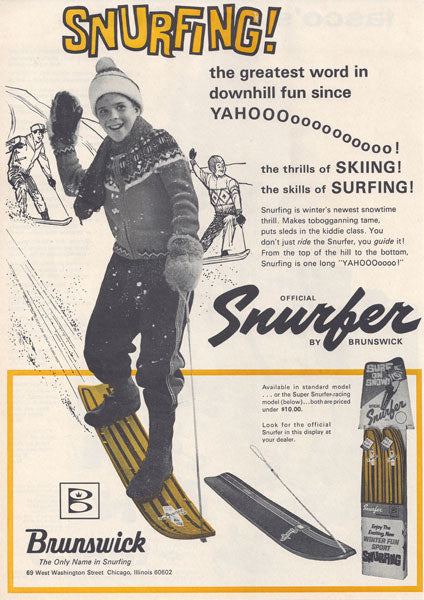This vintage magazine advertisement features a nostalgic, beige-toned background suggestive of old paper. At the top, in large, fun yellow letters accented by a pink backdrop, is the word "Snurfing!" followed by the catchphrase, "The greatest word in downhill fun since Yahoo! The thrills of skiing, the skills of surfing." The ad prominently showcases a black-and-white photograph of a young boy clad in winter attire: a striped sweater, mittens, a scarf, and a wool cap topped with a pom-pom. The boy is joyously riding a snurf board, an early precursor to the snowboard, which tapers to a point at the front. He's gripping a rope handle attached to the snurf board, guiding his descent down the snow-covered slope.

To the right of the boy, snurfing is praised as "winter's newest snow time thrill that makes tobogganing tame and puts sleds in the kiddie class." The text enthuses, "You don't just ride the snurfer. You guide it from the top of the hill to the bottom. Snurfing is one long yahoo!" In the lower corners of the ad are additional images and silhouettes of people joyfully engaged in snurfing, emphasizing the fun and thrill of this winter activity. At the bottom left, the Brunswick logo proudly proclaims it as "Brunswick, the only name in snurfing," cementing its authority and expertise in this exhilarating sport.